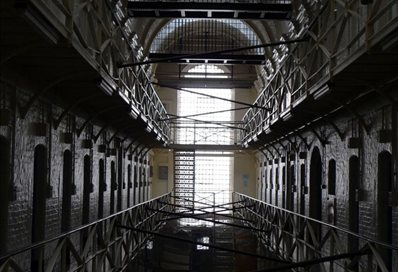The photograph captures the interior of an ancient prison with a distinctly somber atmosphere characterized by its gray and black tones. The image, taken from the second-floor perspective, showcases rows of individual cells, each identified by arched doorways lining both the left and right sides of the walkway. Above each doorway, there are turned-off lights, and beside them, boxes with tubes likely serving as the buzzers for door locks. Enclosed metal railings run along the walkways, designed presumably to prevent inmates from jumping off. The floor is constructed from painted gray brick, adding to the bleak aesthetics of the scene. In the center, metal supports and open metalwork steps connect the different tiers, providing access to the next level. At the far end of the room, a large, two-story window spans the width of the space, adorned with a protective cage and piercing sunlight into the otherwise dimly lit interior. The vibrant light from the window starkly contrasts with the muted shades, highlighting the window's rounded top design that mirrors the doorways. This window also serves as the focal point, providing a glimpse of the elusive freedom beyond the bars.